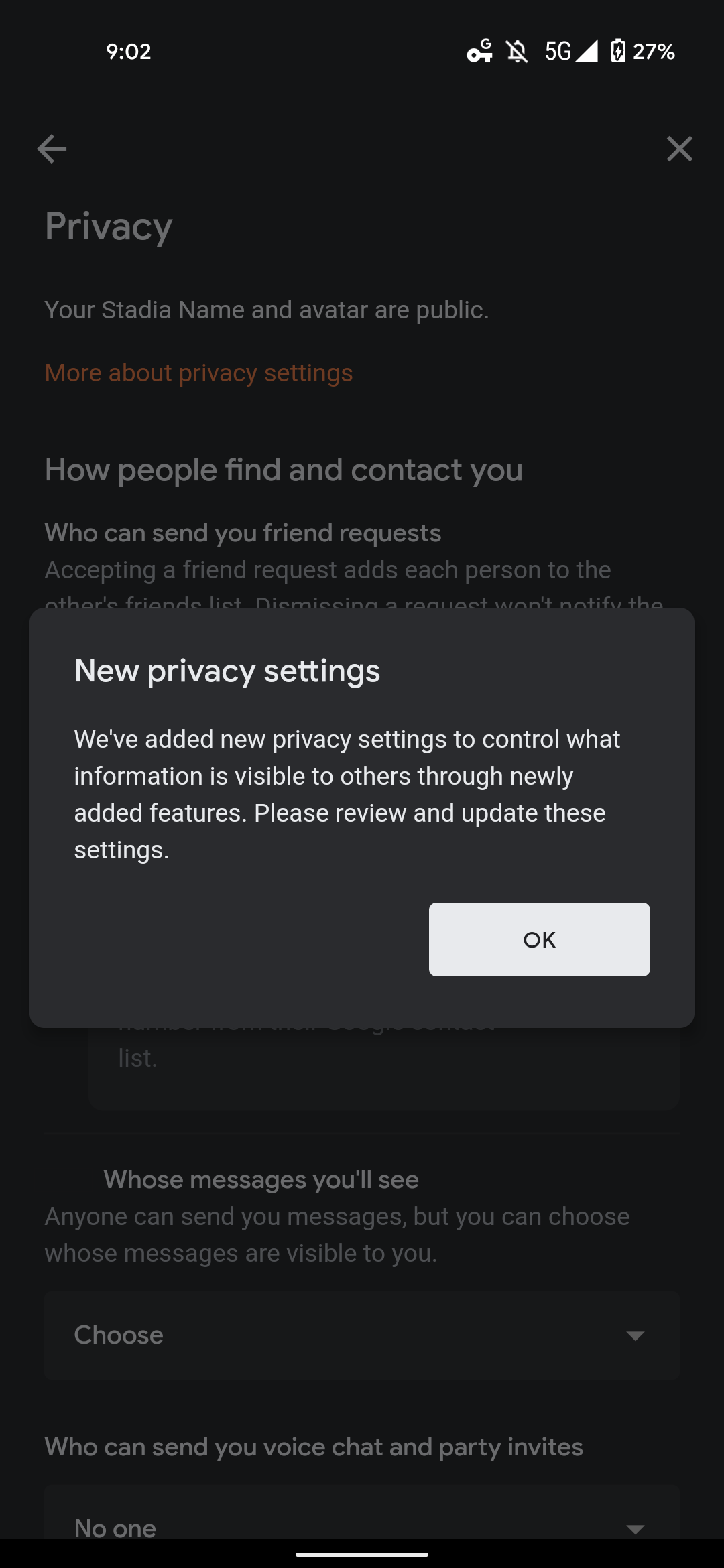The image depicts the Google Stadia privacy policy page, prominently showing a central pop-up message indicating updates to privacy settings. The pop-up highlights that new privacy options have been introduced, allowing users to control the visibility of their information to others. The message encourages users to review and update their settings, featuring an "OK" button to dismiss the notification. 

Behind the pop-up, the privacy policy outlines various settings. At the top, under the heading "Privacy," it notes that your Stadia name and avatar are public. Below, a link titled "More about privacy settings" likely provides further details. Sections on "How people find and contact you," including "Who can send you friend requests," are partially obscured by the pop-up. The visible bottom part of the page includes options for managing interactions, such as "Whose messages you'll see" and "Who can send you voice chat and party invites," each accompanied by a dropdown menu to customize these preferences. The image illustrates the user interface for adjusting contact permissions on Google Stadia.